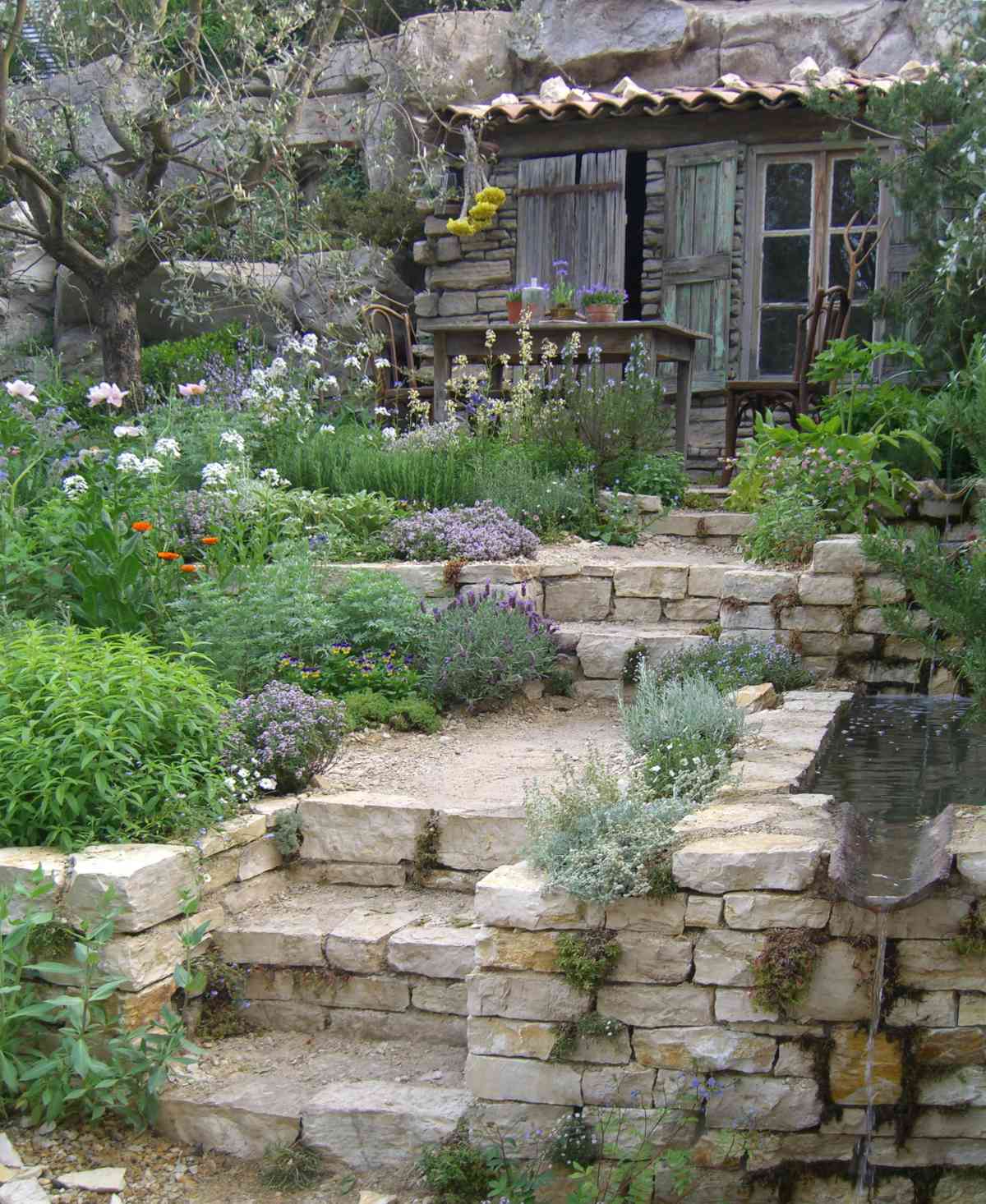The photograph captures a picturesque outdoor scene during the daytime, showcasing a rustic yet vibrant garden setting nestled against a large rock wall. The rectangular image, approximately five inches high by four inches wide, features a multi-tiered stone walkway made from large, light-colored pavers. These steps are interspersed with flat, dirt-covered landings leading the eye upward.

Flanking the steps on both sides are an array of flowering plants in full bloom, creating a tapestry of colors. Small flat purple flowers, taller narrow purple blossoms, white blooms, and a few orange flowers contribute to the lush greenery. Towards the bottom right of the image, a small pool forms the source of a cascading waterfall that flows gracefully down the side.

At the top of the steps, embedded into the rock wall, is the front facade of a wooden cabin. This quaint structure features a window, wooden shutter doors, and a tiled roof. In front of the cabin, a wooden table with matching chairs is set out, adding a touch of homeliness. Clay pots filled with purple flowers adorn the table, while red flowers dangle from the cabin’s covered porch.

To the left part of the photograph, a grand tree stands tall, completing the serene environment. The entire scene melds rugged natural elements with cultivated beauty, presenting a harmonious blend of stone, flora, and water features. The overall effect is a beautiful garden oasis, rich in color and detail.